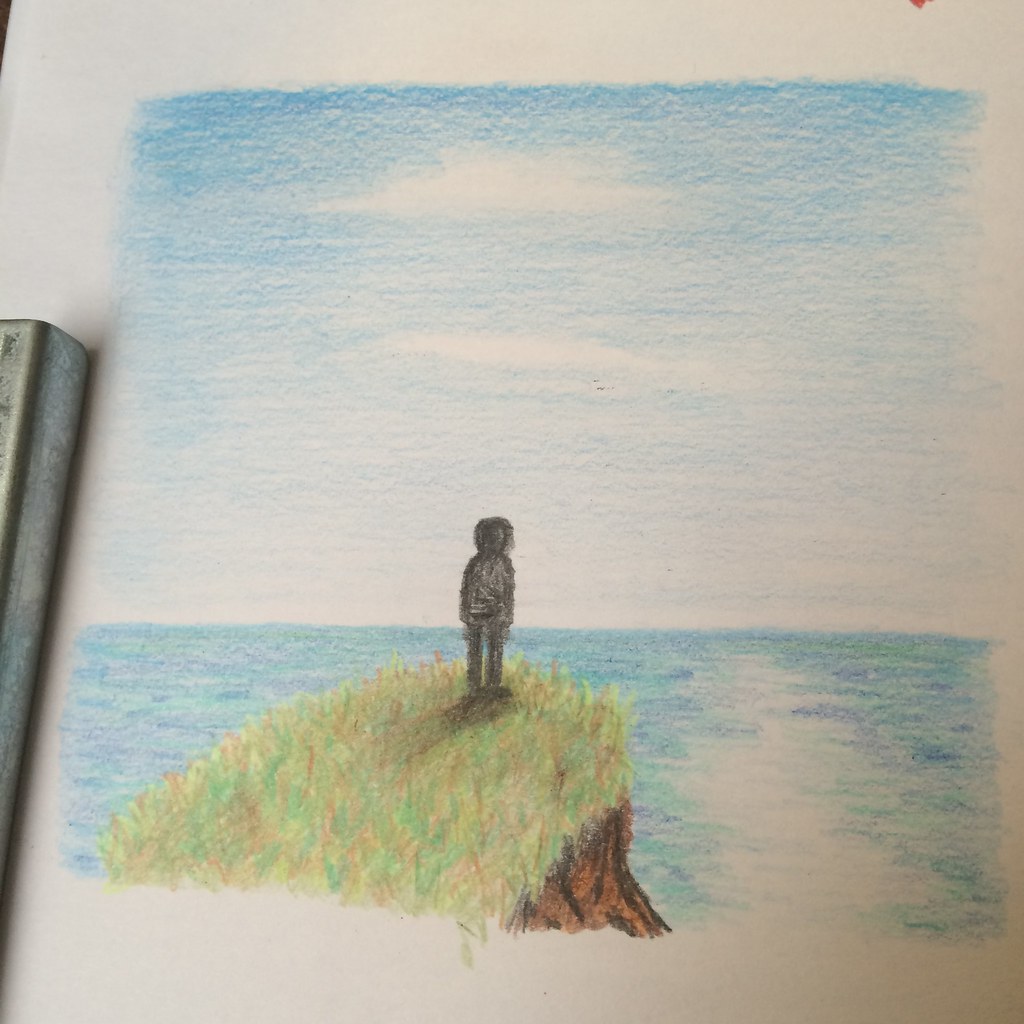The photograph captures a vibrant, hand-drawn illustration created with color pencils, showcasing a picturesque scene. The drawing depicts a silhouette of a person standing on a small, projecting hillside overlooking the ocean. The water is intricately colored with a blend of blues, turquoises, and purples, featuring a delicate reflection stretching across the right side of the water, thinning toward the horizon. Above, the sky transitions from a deep blue at the top to almost white near the horizon, punctuated by a few fluffy white clouds. The outcrop on which the person stands is covered in lush green grasses, interspersed with browns and yellows, suggesting a mix of tall weeds and shorter grass. The base of the hillside shows hints of brown soil, and the illustration ends abruptly in the bottom right corner of the paper.